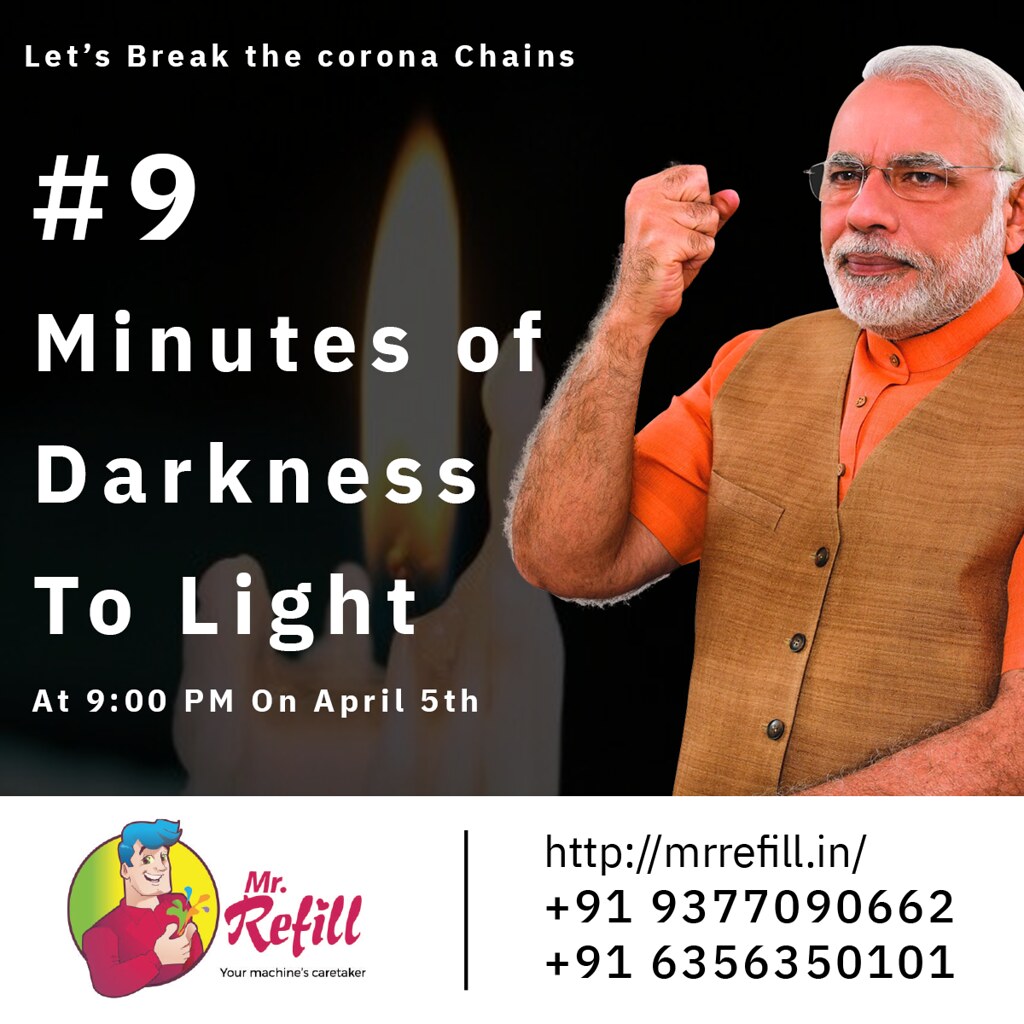The image is an informational card or poster predominantly featuring a man with a serious expression on his face. The top 80% of the card shows the man facing forward and slightly to the left, his right fist raised in the air. He has short white hair, a white beard, and a mustache, and he wears glasses, a tan vest over a bright orange shirt. The background is black, with a large candle flame visible behind him. In large white letters on the top left side, the text reads: "Let's Break the Corona Chains. #9. Minutes of Darkness to Light." Following that, it states, "at 9 p.m. on April 5th." At the bottom portion of the card, an ad for Mr. Refill is displayed. This includes a vertical black line separating an image of a cartoon man with blue hair and a red shirt inside a yellow circle on the left and the text "Mr. Refill, your machine's caretaker" on the right. Below the ad, there is a URL: "http://mrrefill.in/" followed by two long numbers in black text.